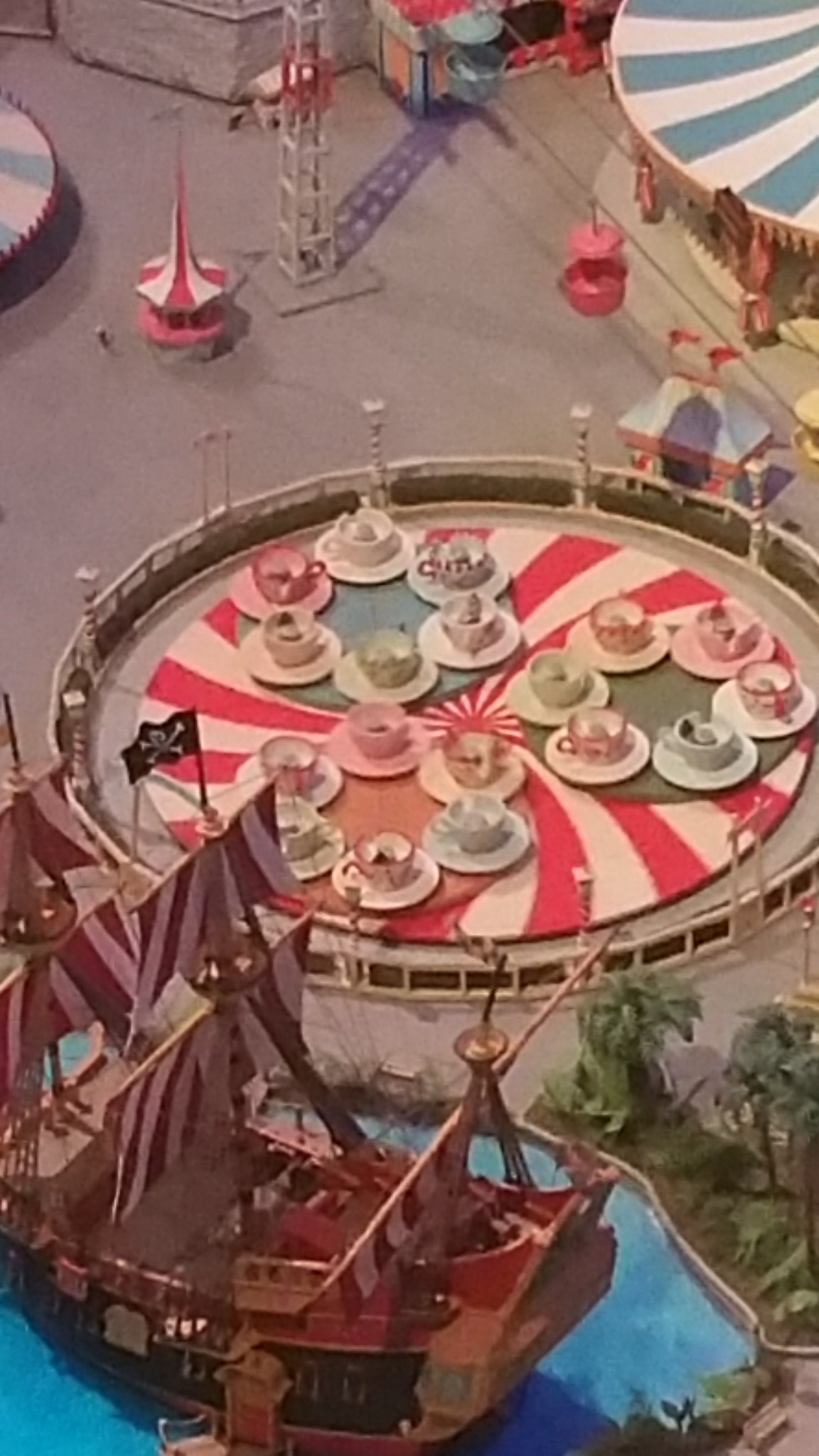The image appears to be a highly detailed, top-down illustration or concept art of a theme park, reminiscent of a toy carnival setting. Dominating the center is a vibrant teacup ride, featuring a large circular platform adorned with a hot pink and white swirl pattern. Surrounding the edge of this platform are three smaller circles, each hosting six teacups in alternating colors of blue, green, yellow, and pink. The teacups are occupied by people, indicating it as a live attraction. 

Encircling the teacup ride is a low, white fence intermittently topped with posts bearing white lights, contributing to the festive atmosphere. To the lower left, nestled in an oval-shaped body of bright blue water, is a grand pirate ship with tan hulls and red-striped sails. The ship is adorned with a small black Jolly Roger flag and is accompanied by palm trees lining the right of the water.

On the upper right side of the image stands a majestic carousel housed under a large circus tent accented with white and blue stripes. The upper left corner features another circular structure, while the top of the image is filled with a stretch of featureless gray concrete, interrupted occasionally by stands and kiosks. One notable kiosk to the left showcases a painted pink and white umbrella. The illustration captures the bustling, colorful, and detailed essence of a lively theme park.